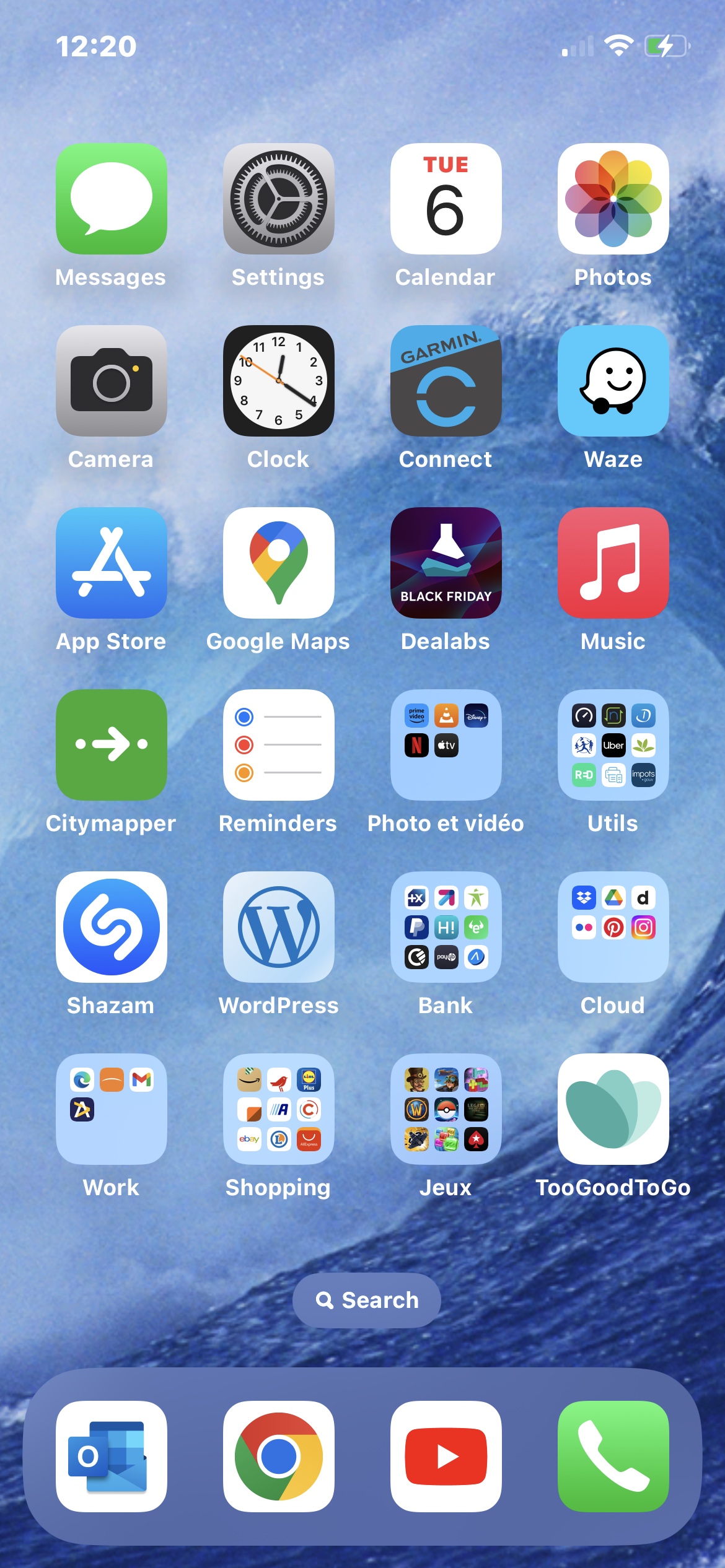This image depicts a smartphone screen with a vibrant and dynamic background featuring a giant wave curling into the left side of the screen. At the top of the screen, the usual status indicators are present: the current time displayed in the upper left corner, minimal phone signal strength, a Wi-Fi connection symbol, and a charging icon. 

The lower part of the screen contains four persistent app icons: Phone (for making calls), YouTube, Chrome, and another one that resembles iTunes. 

The main section of the screen displays 24 app icons, neatly arranged in a grid pattern. These apps include Messages, Settings, Calendar, Photos, Camera, Clock, Connect, Waze, App Store, Google Maps, D-Labs, Music, Citymapper, Reminders, Photo & Video, Utils, Utilities, Shazam, WordPress, Bank, Cloud, Workshopping, ZHU, and Too Good To Go. Some of these icons represent folders that contain multiple apps, such as Utils, Photo & Video, and Bank.